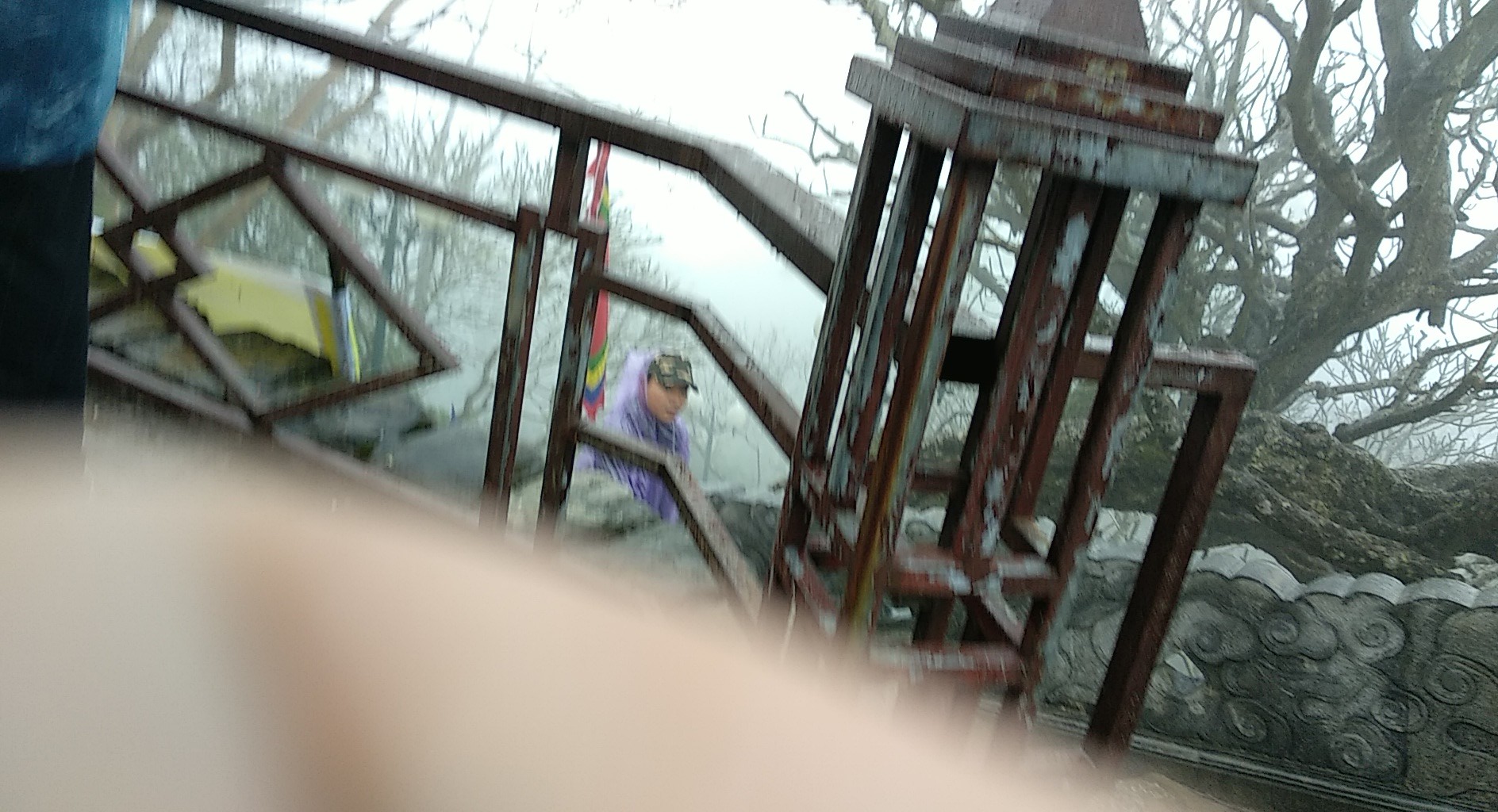In this blurred, low-resolution photograph, possibly digitally enhanced, we see a section of an outdoor stairwell situated in what appears to be a park. The focal point is an iron gate featuring geometric shapes, with a diamond pattern stemming from the ground and a rail on top. Beneath the rail, there is a person either sitting or standing as if ascending the stone stairs, which are set horizontally from the upper left to the lower right of the image. This individual, only visible from the waist up, is dressed in a blue shirt or jacket and a cap, with fair skin. The background showcases a line of leafless trees extending from the upper left to the lower right. The lower left corner of the image contains an indistinct, light tan blur, the specifics of which are unidentifiable.